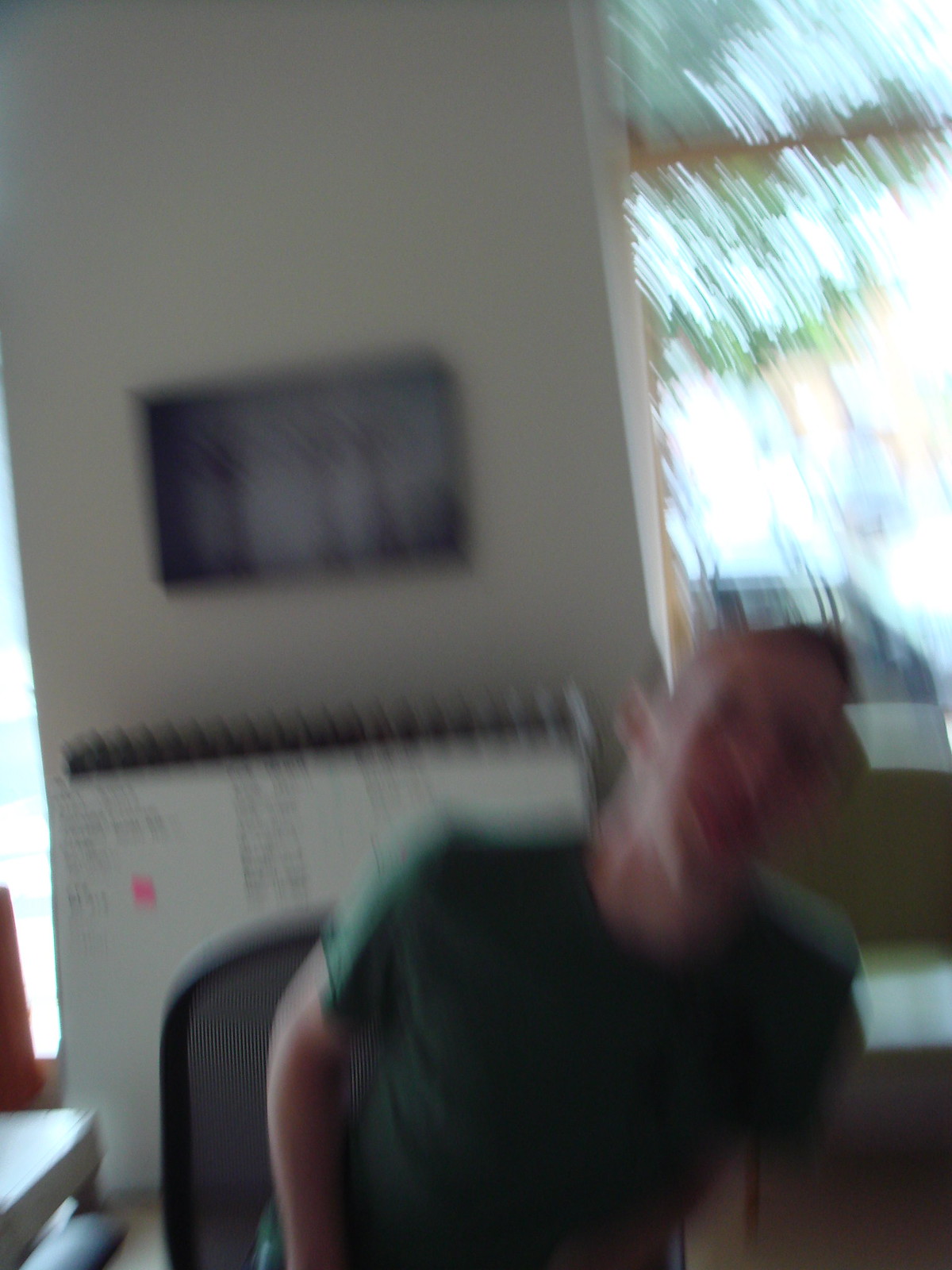In this photograph, a man is sitting in a black chair inside a room. He is wearing a short-sleeved green t-shirt and is tilting slightly towards the left, facing the camera, although his face is too blurry to make out any details. Behind him, a window allows light to filter into the room, suggesting the presence of a tree outside, as indicated by the green hues visible through the glass. The adjacent wall is painted gray and features a square picture hanging on it. Below this picture, there is a white chart with a black top, leaning against the gray wall. No curtains are visible on the window, adding to the softly-lit, indistinct atmosphere of the image.